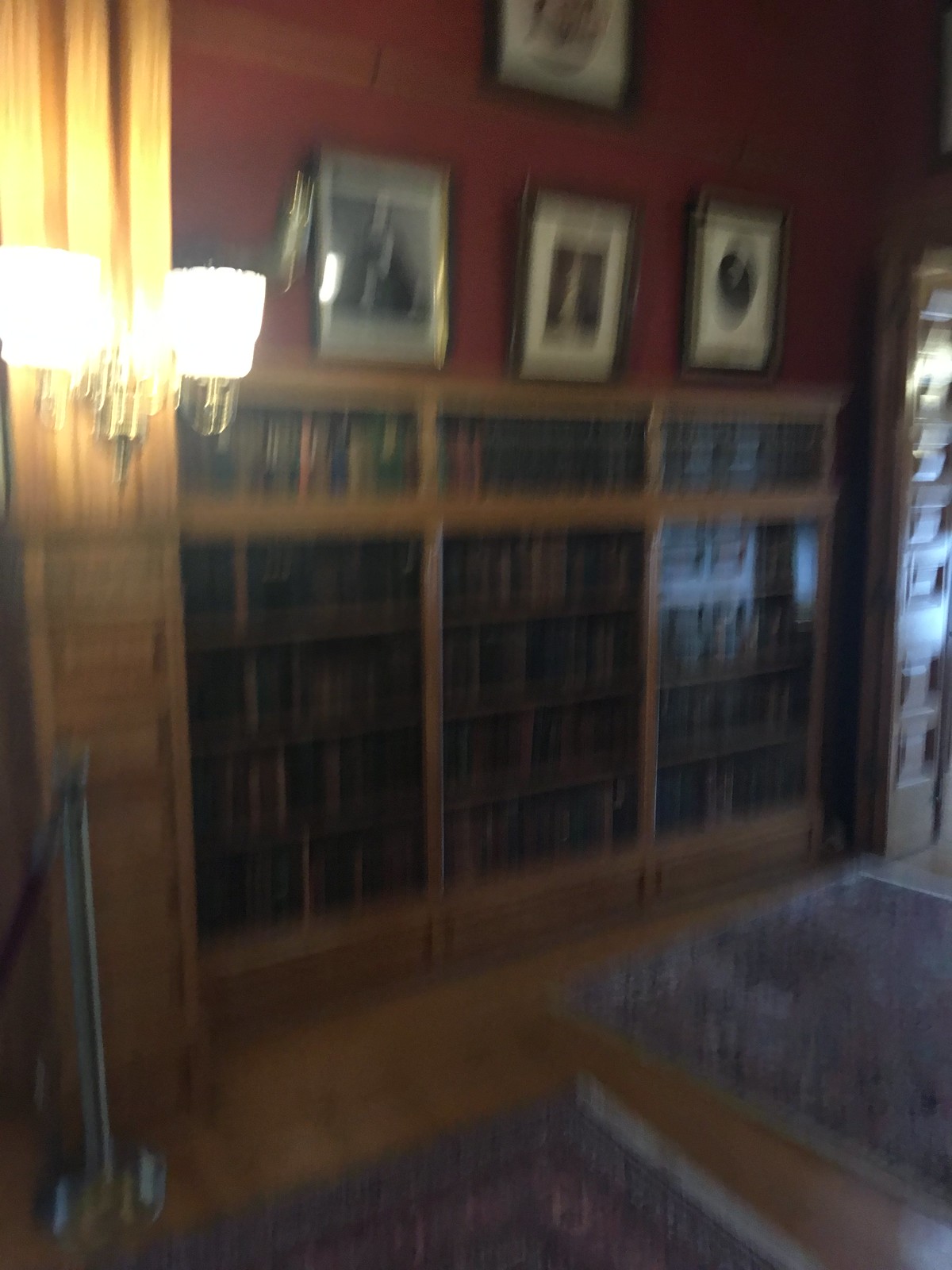An indoor photo captures a cozy, dimly lit library space within a residential setting. The image, slightly out-of-focus, showcases an ambiance of warmth accentuated by wooden floors and wooden trim adorning the walls. Central to the scene is a substantial wooden bookcase partitioned into three sections, each filled with an assortment of books. The bookcase features five shelves in total, with the top shelf demarcated by a prominent line, and the remaining four shelves offering open space for various titles and decor. Above the bookcase are three framed photographs positioned in a neat row, with an additional photograph placed above them. The frames are either black or wood-toned, contrasting beautifully against the rich, red-painted wall.

The floor is adorned with two oriental rugs, adding to the room’s inviting and elegant atmosphere. To the far right, a metal rack, possibly for magazines, introduces a touch of modernity to the otherwise traditional decor. A metal bar with an attached rope stands nearby, perhaps serving as a guide or a standing area marker. Overall, the scene exudes a blend of classical charm and comfort, inviting one to linger and explore the literary collection.